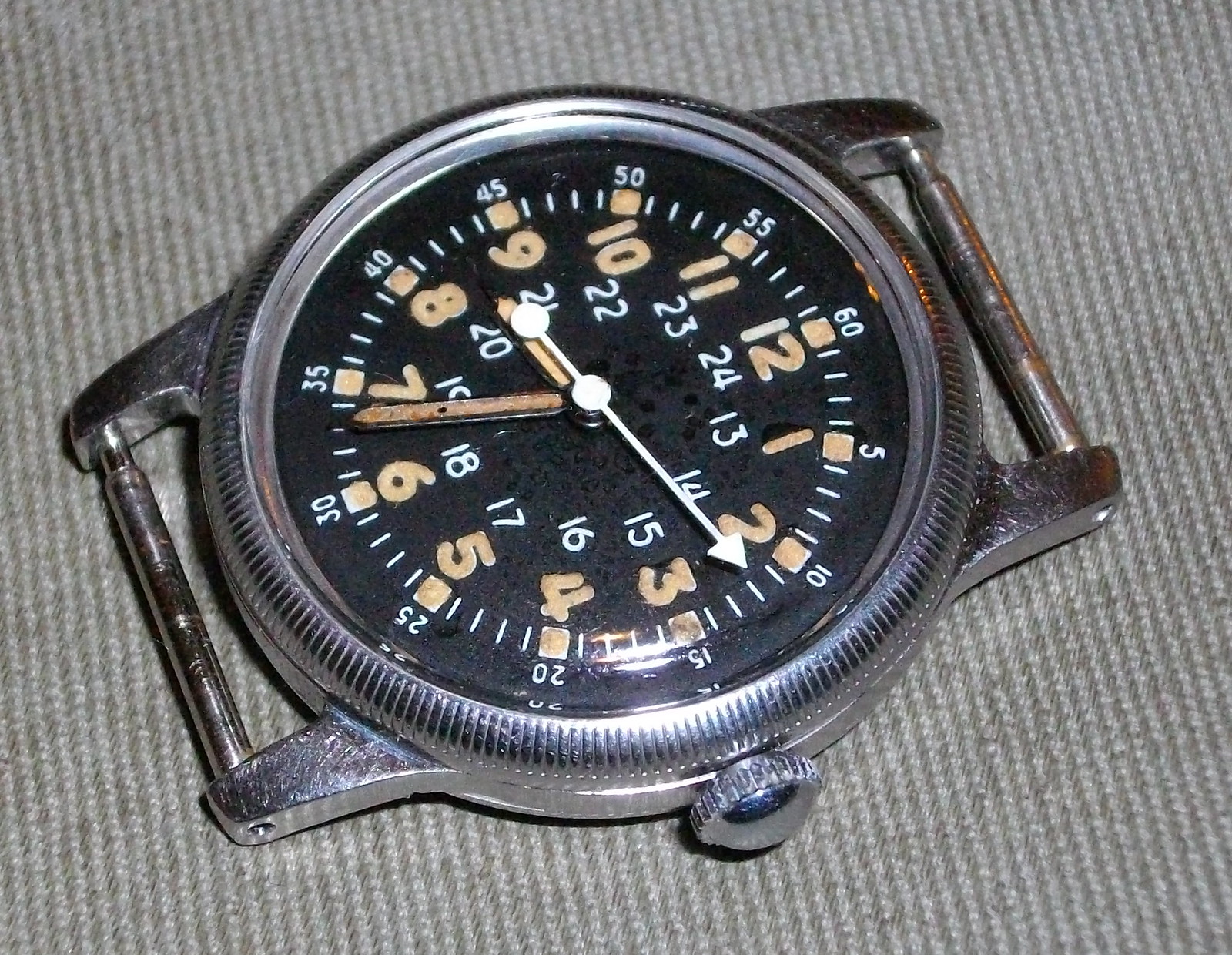This image features a vintage 1956 Waltham mechanical watch, showcasing only the watch face without any straps. The timepiece, made of silver or stainless steel, exhibits signs of age with a bit of rust on the sides and a surface speckled with black marks. The face itself is black, adorned with large, orange-pinkish numerals for the hours, encircled by smaller white numerals for military time (13 to 24 hours). The seconds are marked in intervals of five along the outer edge, from 60 above the 12 down to 5 above the 1. The watch hands, while slightly discolored and rusty, remain white, with a more vibrant longer hand compared to the shorter. The background appears to be a textured gray carpet with darker and lighter strips, possibly under shadows, providing a contrasting backdrop to the silver-rimmed watch, which lies slightly tilted on its side.